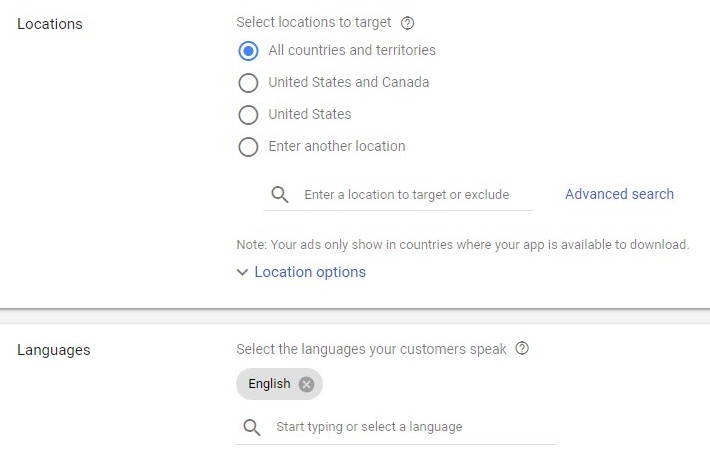In the image, there is a white background with greyish font. On the left side, the word "Locations" is displayed, and to its right, it reads "Select Location to Target." Adjacent to this is a grey circle with a grey question mark inside. Below this are four circles: the first circle is blue-outlined and white, with another blue circle in the center. To the right of this first circle, it says "All Countries and Territories."

The first line below the grey circle says "United States and Canada." The next grey circle below that says "United States," and to the right of it, another grey circle states "Enter Another Location." Just slightly to the right of this is a search icon (magnifying glass), and next to it are the words "Enter a Location to Target or Exclude." To the right, in what appears to be blue font, it says "Advanced Search."

Beneath the "Enter a Location to Target or Exclude" text is a grey line, followed by a note that reads: "Note: Your ads only show in countries where your app is available to download."

Further down on the left is a grey arrow pointing downwards, followed by the text "Location Options" in blue font. There is a darker grey line and a light grey square underneath this. Moving to the left again, it says "Languages." To its right, there are the words "Select a Language Your Customers Speak," accompanied by a grey circle with a grey question mark inside. Next to this is another faded grey circle, next to which, in black font, the word "English" is displayed along with an 'X' in a darker grey circle.

Underneath this is another magnifying glass icon, and next to it, the text "Start typing or select a language." Below this is a grey line.